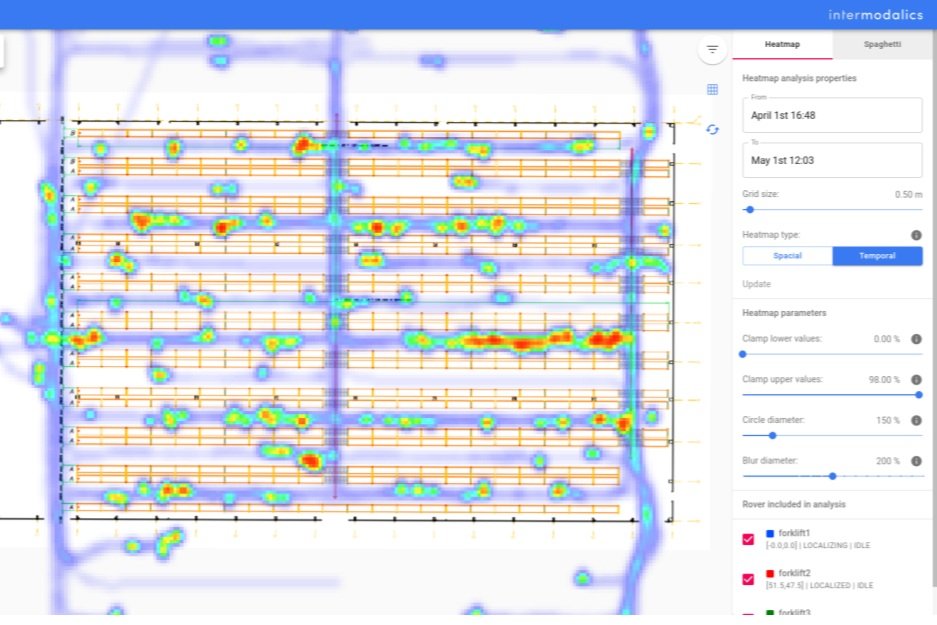This screenshot showcases a results page with an intricate heat sensor overlay. The top of the screenshot features a gradient of light to medium blue, with "Intermodalics" prominently displayed in the top right corner. The central part of the image, occupying roughly two-thirds of the screen from left to right, features an orange grid overlay that resembles an infrared heat map. Various lines within the grid transition in color from blue to dark red, indicating different heat levels. Along the bottom or within the grid, the dates "April 1st to May 1st" are legible, though other text remains too small to decipher. The background also includes a patterned grid of purple lines, which further integrates heat sensor data in specific areas, adding layers of complexity to the visual representation.